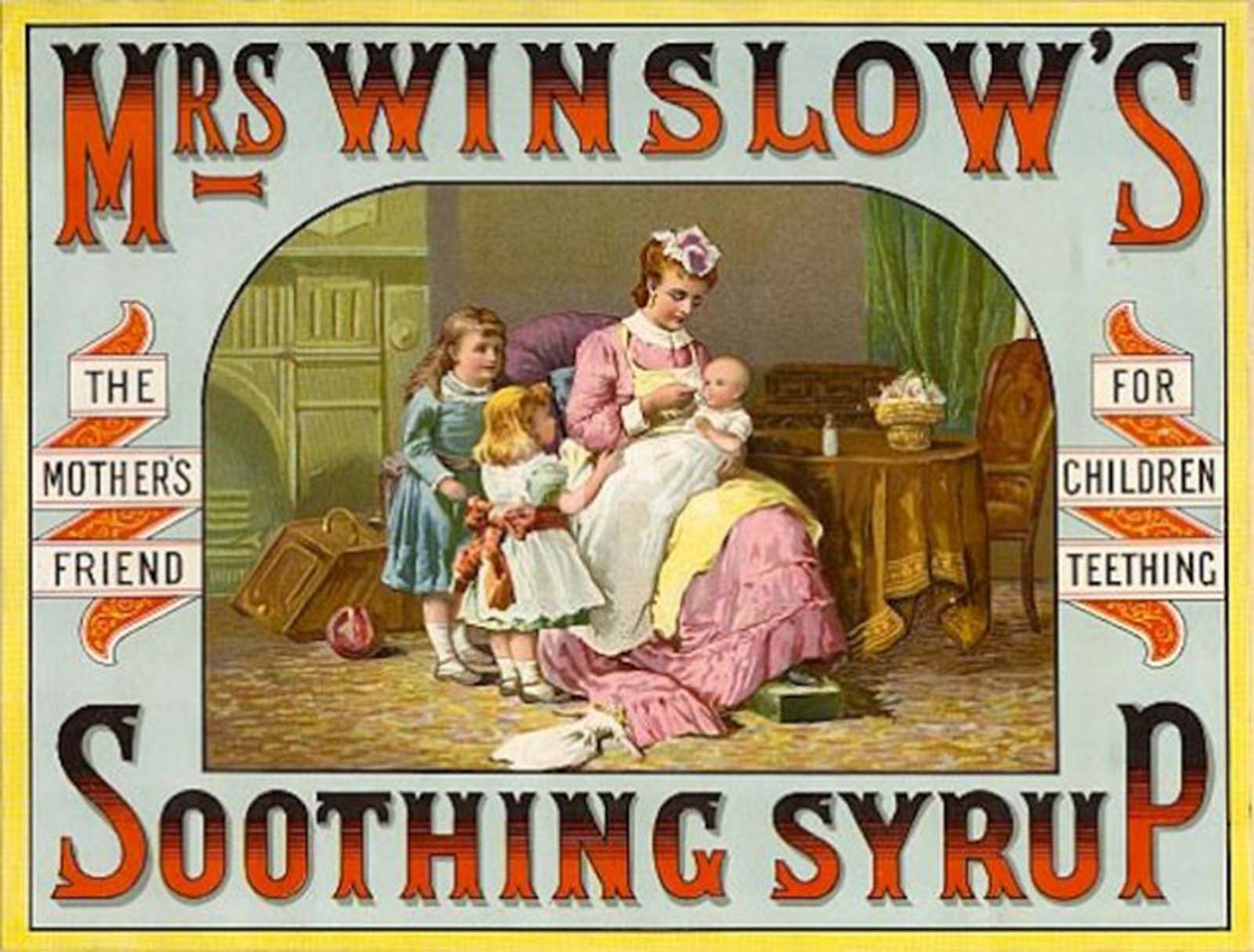This vintage advertisement for Mrs. Winslow's Soothing Syrup, a medication for teething children, features a horizontally aligned rectangular image with a gold-colored border and a thin black inner border. At the top of the advertisement, "Mrs. Winslow's" is printed in large, distinctive letters, with the 'M' in the upper left corner and the 'S' in the upper right corner, both larger than the rest. Similarly, at the bottom, "Soothing Syrup" is written with the 'S' in the lower left corner and the 'P' in the lower right corner, also larger. On the left side, vertically printed in white rectangles with black text, it reads "The Mother's Friend," and on the right, "For Children Teething." 

The central artwork, outlined in black, depicts a nurturing mother in a long, Victorian-style pink dress with a white apron, sitting in a living room near a fireplace to the left and a sitting table. She has orange-colored hair and a yellow blanket over her lap, and is depicted feeding a baby with a spoon. The baby sits in her lap while two small toddlers stand beside her, completing this warm, familial scene.